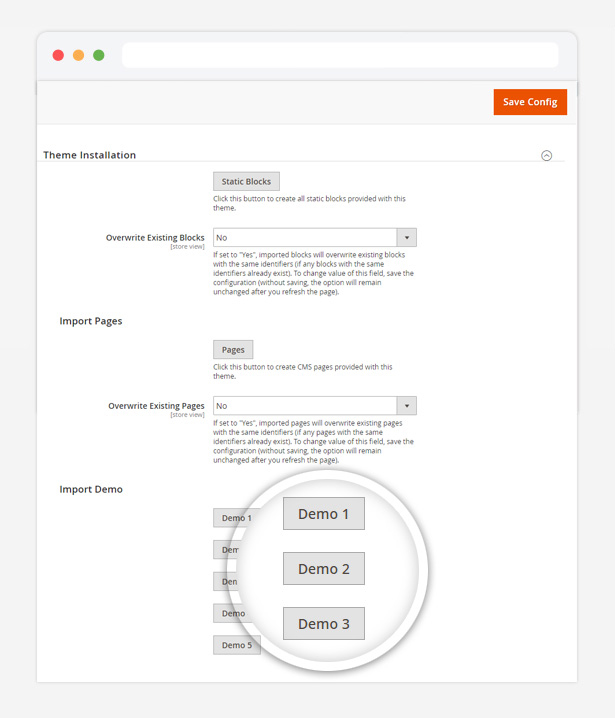The image appears to be a screenshot from a web or app interface that is likely part of an Apple MacBook setup, given the familiar design elements. The background is grey, overlaid by a white window located centrally. The window has three circular buttons on the upper left corner: one red, one yellow, and one green, characteristic of macOS design.

On the top portion of the window, beside the colored buttons, there's an empty search bar. Further below, on the right side, a prominent red button labeled "Save Config" with white text is displayed. To its left, the text "Team Installation" is clearly visible in black.

Below this, there's a section labeled "Static Blocks" in a grey box with black text. This section includes a button for creating all static blocks provided with the team, and a dropdown menu labeled "Overwrite Existing Blocks, Store View" with the default selection set to "No." When set to "Yes," options to import or overwrite existing blocks with the same identifiers are enabled.

The "Import Pages" section follows, containing a similar setup—a button to create CVS pages provided by the team and a dropdown menu for "Overwrite Existing Pages, Store View" set to "No." Like the static blocks, setting this to "Yes" will allow overwriting pages with the same identifiers upon saving the configuration.

On the left side, the "Import Demo" section is visible, displaying a list of demos. One demo is clearly visible at the top, with five additional demos partially shown below. There is a distinctive circular magnifying tool on the right side that helps to enlarge the list. This circle has two outer white bands, and inside, it contains three large grey rectangles stacked vertically, labeled "Demo 1," "Demo 2," and "Demo 3."

Overall, the interface seems to provide options for managing static blocks, pages, and demos, with various configuration settings accessible through dropdown menus and buttons.